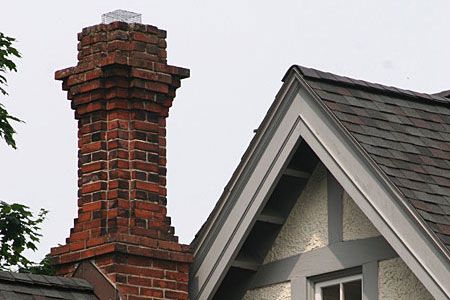The image captures a somewhat overcast day with a gray, cloudy sky. Dominating the scene is a brick chimney, composed of aged red and black bricks, which stands atop the roof of a house. The chimney has a silver metal grate at the top, likely placed to prevent birds and other debris from entering. The roof of the house consists of gray and black shingles. To the left of the chimney, a tree with green leaves extends into the frame. The house itself features a white facade with gray trim along the roofline and has a distinctive popcorn texture underneath the roof’s overhang. There's also a mention of blue trim around the windows, adding a splash of color to the otherwise monochromatic theme. The overall aesthetic gives the impression of an older, weathered chimney juxtaposed against a relatively newer-looking house, providing an intriguing contrast.